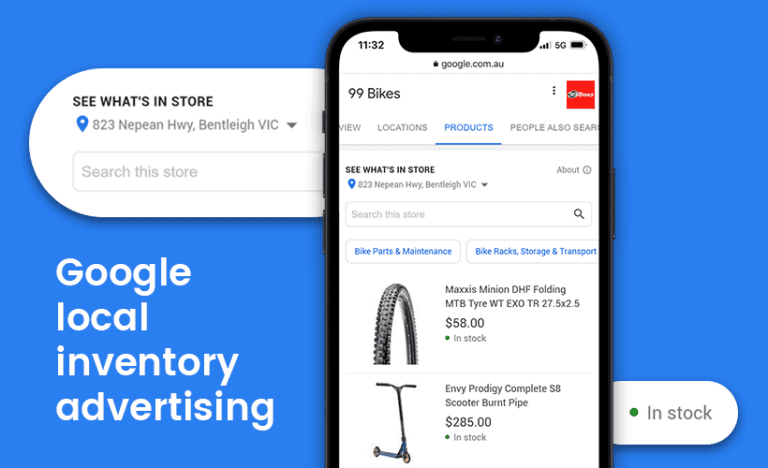In the image, the backdrop is a serene blue. Positioned towards the center-right is a sleek smartphone featuring a black bezel. Surrounding the smartphone are various textual contents.

On the top left of the image, there is a black text on a white background that reads, "See what's in store". Below this, the store's location is specified as "823 NEPAN HWY BENTLEY VIC". Adjacent to this section is a search button labeled "Search the Store". Beneath this, in white text positioned at the lower left, is the phrase "kukli local inventory advertising". 

On the bottom right, the words "In Stock" are prominently displayed next to a green dot. On the smartphone's screen, the URL "kukli.com.au" is visible. Below the URL, a search bar contains the text "99 bikes" with a red accent to the right of the search bar.

Underneath the search bar, various terms are listed: "View Location," "Products," and "People Also Search." The term "Products" is highlighted. Below this, the text "See what's in store 823 NEPAN HWY BENTLEY VIC" appears once again. Directly underneath is another search button that says "Search the Store".

Further down, there are categories written in blue for "Cycling", "Bike Parts and Maintenance", and "Bike Racks Storage and Transport". Below these categories, there are images of two products:

1. "MEXIS MINION DHF Folding MTB Tyre WT EXO TR 27.5x2.5" priced at $58, noted as in stock. The tyre is black.
2. "ENVE PRO DIGICOMPLETE SA Scooter Bent Pipe" priced at $285, also marked as in stock.

The entire composition of the image effectively details the online store's offerings and provides a navigational guide to potential customers.